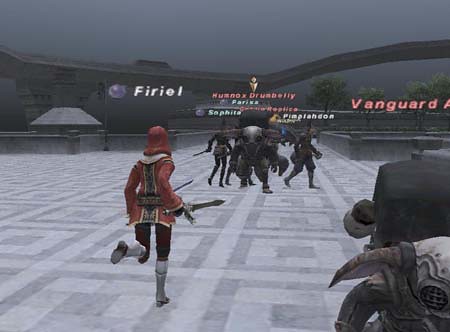The image is a screenshot from a video game showcasing a dynamic combat scene in an open cement courtyard with a dark gray, cloudy sky. The ground features a tiled pattern of white and gray squares. In the bottom left, a character is captured mid-run with their left foot in the air and their right foot firmly on the ground. This character is notably dressed in black pants, knee-high silver boots, and an elaborate red and gold tunic with a red hood over a white collar. They wield a sword in their right hand. Ahead of this character, there is another figure with horns and various monster-like entities on either side suggesting a battle scene. Above the heads of these characters, there are neon signs and usernames in different colors, such as "Firell," "Drumbelly," "Huznox," and "Fariel." To the right side of the image is a gray square with another horned being. The background reveals what appears to be a bridge or roof structure along with some distant trees, adding to the intricate and thrilling atmosphere of this in-game world.